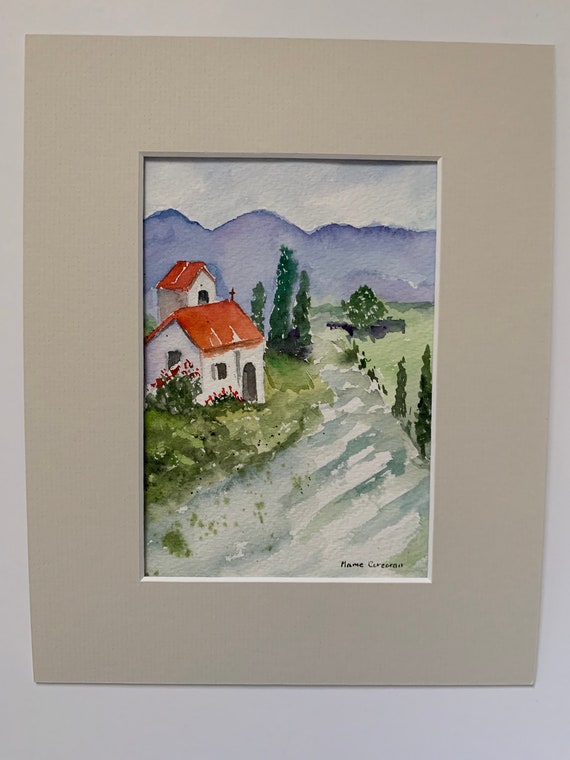This image is a detailed watercolor painting of a quaint village scene featuring a small white church with a red roof and a prominent cross atop its arched doorway. The church is set amidst charming greenery, including evergreen trees and red flowering bushes, which line a gray country road that fades into the background. Adjacent to the church stands another building, also white with a matching red roof, which could be associated with the church. The artwork captures a serene landscape with light blue skies and purple mountain ranges in the background, adding to the picturesque tranquility of the scene. The painting, artistically bordered with tan mounting and yet to be framed, is signed by an artist whose first name appears to be Mame or Mamie.